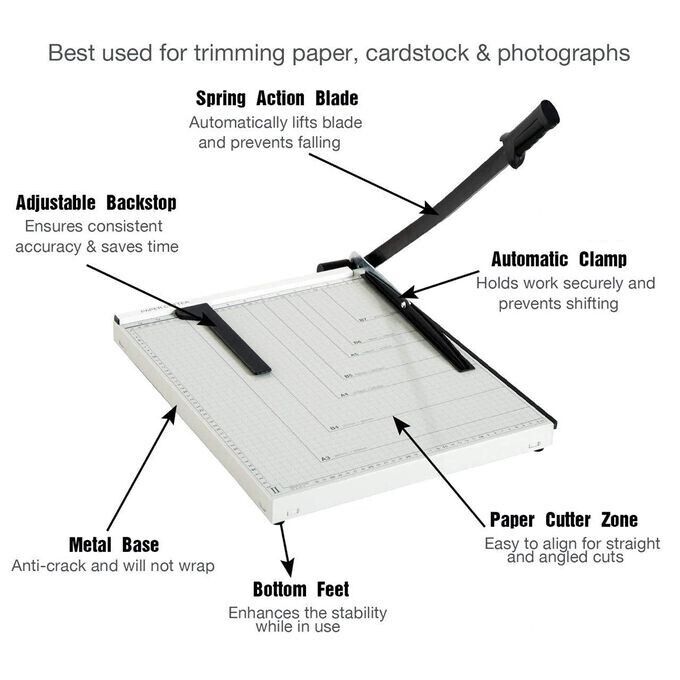This detailed illustration showcases a high-precision paper cutting machine, designed primarily for trimming paper, cardstock, and photographs. The predominant white base of the cutter features a comprehensive grid system with clear black lines and text, making it user-friendly for aligning straight and angled cuts. At the heart of the cutter is a spring action blade on the right side, resembling a sword with a black handle, which automatically lifts and prevents accidental falling. An adjustable backstop slides across the top, ensuring consistent accuracy and saving time. The metal base is constructed to be anti-crack and warp-resistant, and stability is further enhanced by bottom feet that prevent slipping. An automatic clamp also holds materials securely, preventing any shifting during use. Labeled clearly, each feature reinforces the machine's efficiency and reliability, making it an essential tool for precision cutting.